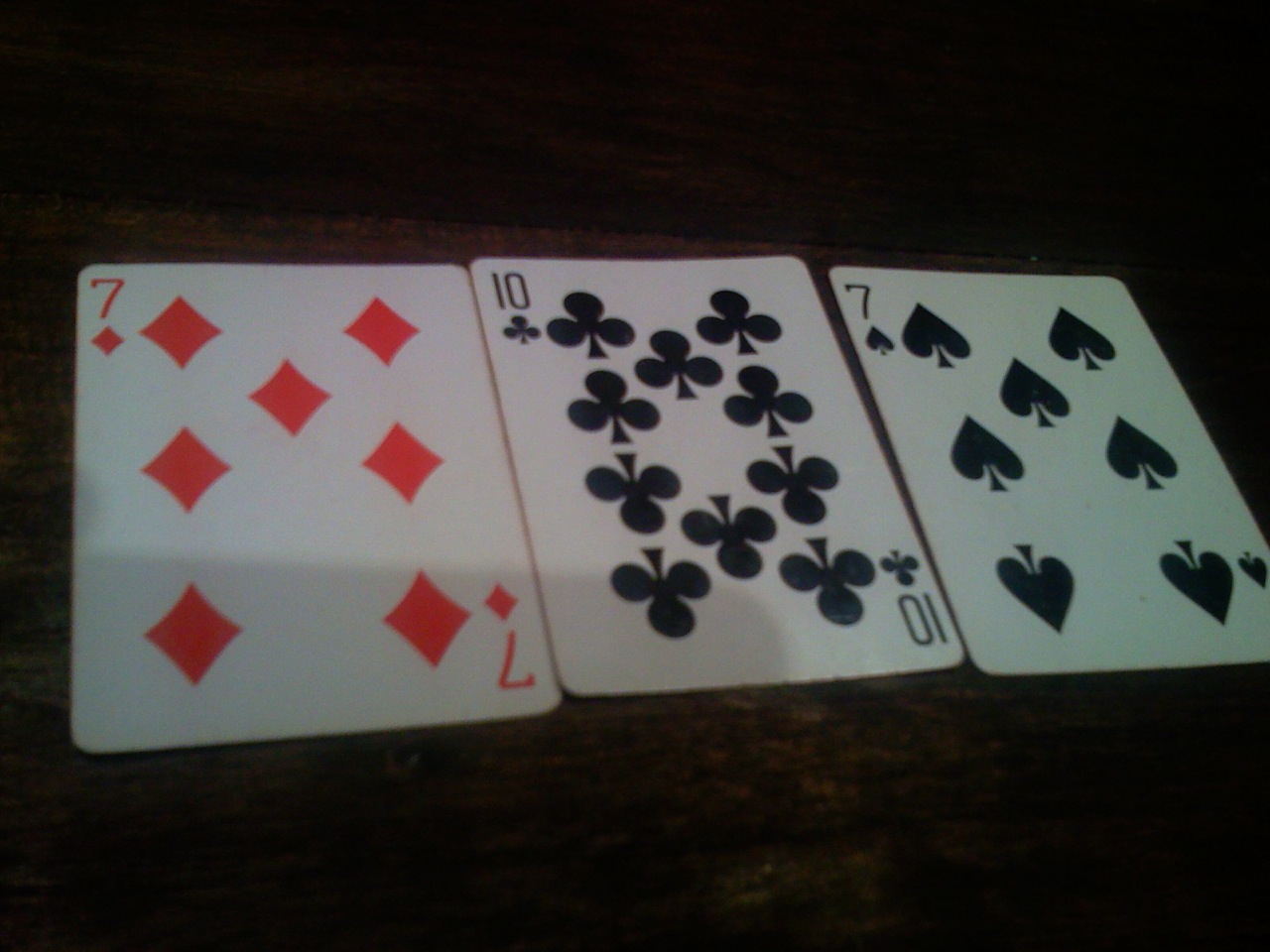In the image, three playing cards from a standard deck are arranged side by side. On the far left is a red seven of diamonds, followed by a ten of clubs in the center, and a seven of spades on the far right. The colors of the cards, from left to right, are red, black, and black. The background is partially visible and appears to be a wooden table, though the image is slightly underexposed, making it difficult to confirm. Additionally, in the bottom left-hand corner, there is a noticeable shadow, possibly cast by a camera or phone belonging to the person taking the picture, obscuring part of the light source.